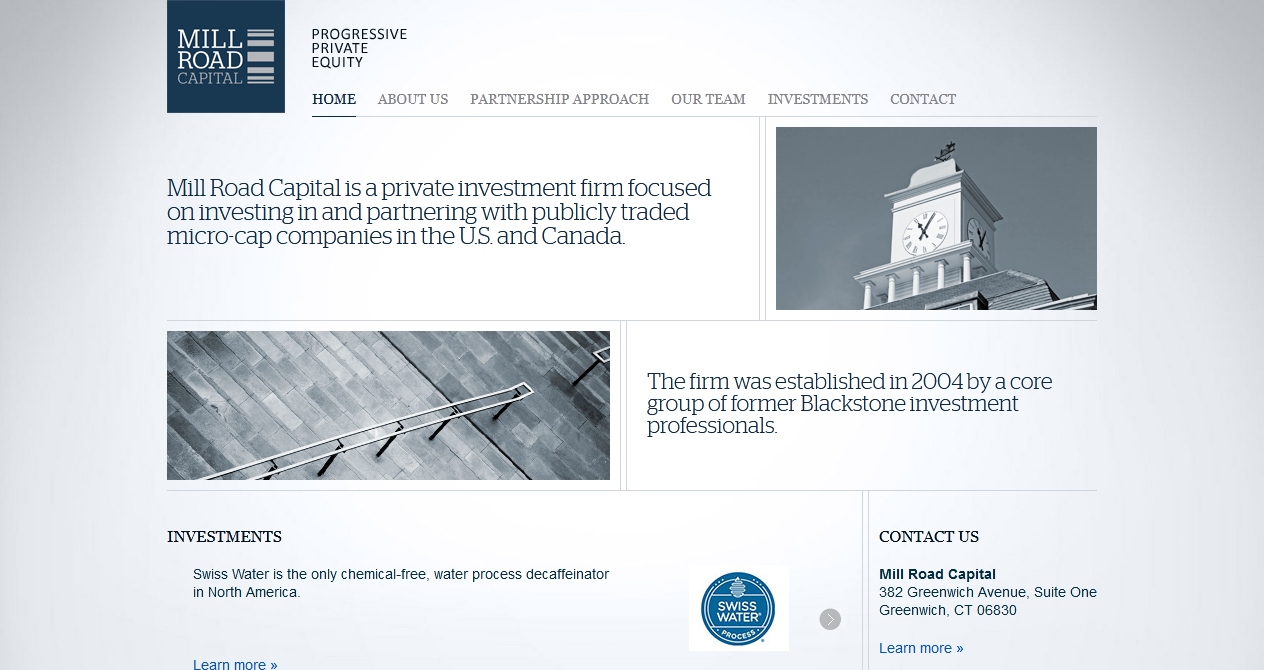This is a detailed screenshot of the web page for Mill Road Capital. In the upper left-hand corner, a square black box with white text prominently displays the company name, "Mill Road Capital." Adjacent to this box, the tagline "Progressive Private Equity" is clearly visible. The top navigation bar offers options for "Home," "About Us," "Partnership Approach," "Our Team," "Investments," and "Contact."

Beneath the navigation bar, the left section contains a rectangular block of text that introduces the firm: "Mill Road Capital is a private investment firm focused on investing in and partnering with publicly traded micro-cap companies in the U.S. and Canada." 

To the right of this block of text is another rectangular section featuring a central photograph of a clock tower, which displays the time "11:05."

Lower in the center of the screenshot, there is a rectangular image of concrete or brick stairs, complete with a metal railing on the right side.

To the right of this photograph, text details the company's origins: "The firm was established in 2004 by a core group of former Blackstone investment professionals."

At the bottom, the page highlights one of their specific investments: "Investments, Swiss Water is the only chemical-free water process decaffeinator in North America." Accompanying this text is a blue circular logo for Swiss Water.

In the lower right corner, the Contact Us section provides the company's address: "Mill Road Capital, 382 Greenwich Avenue, Suite 1, Greenwich, Connecticut, 06830."